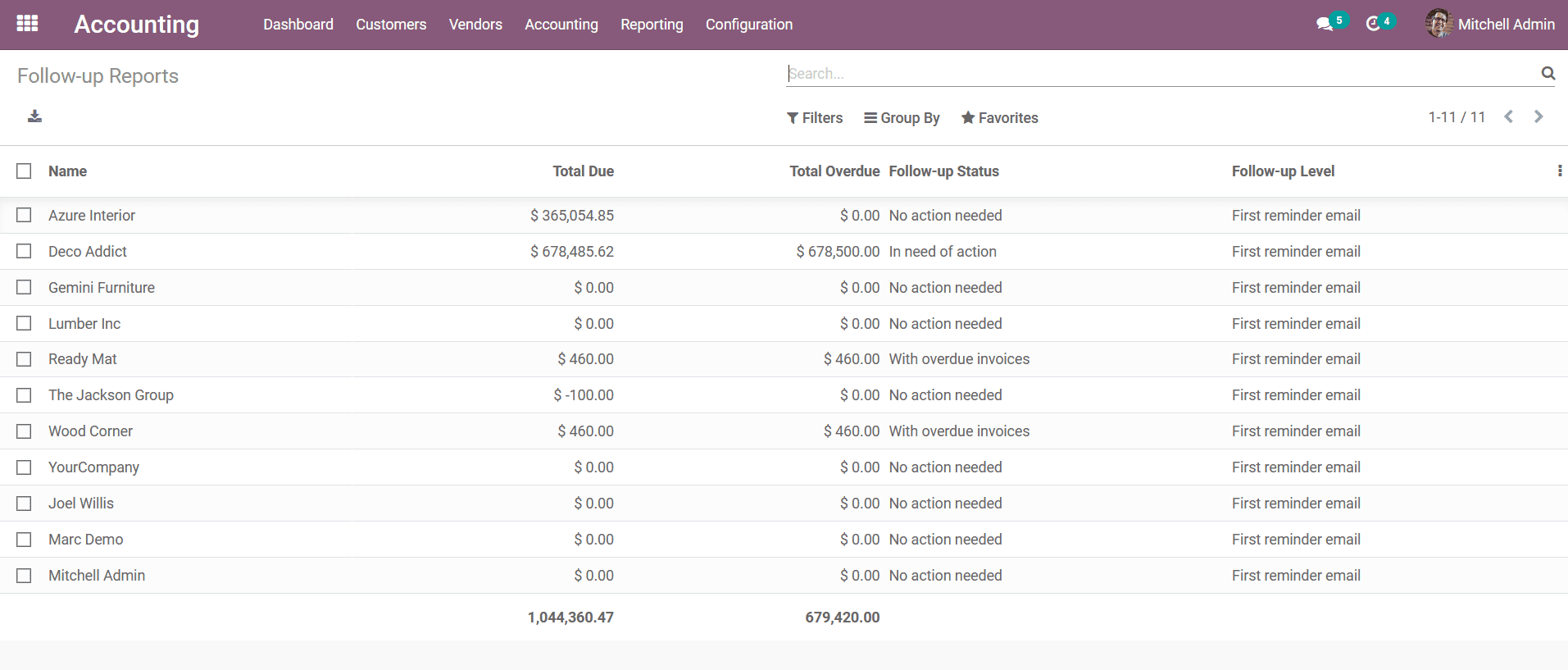The webpage displayed is an accounting dashboard with a light maroon or plum-colored top bar. The bar features a small square icon consisting of nine smaller boxes, and it offers a navigation menu with the following options: Dashboard, Customers, Vendors, Accounting, Reporting, and Configuration. Additionally, the user has five messages or notifications, and the page identifies the user as "Mitchell Administration."

Below the navigation bar is a section titled "Follow-up Reports," which is organized into four categories: Name, Total Due, Total Overdue, Follow-up Status, and Follow-up Level. The entries include:

1. **Azure Interior**:
   - Total Due: $365,000+
   - Total Overdue: None
   - Follow-up Status: No action needed
   - Follow-up Level: First reminder email

2. **Deco Addict**:
   - Total Due: $678,000+
   - Total Overdue: Entire amount
   - Follow-up Status: Action required
   - Follow-up Level: First reminder email

3. **ReadyMap**:
   - Total Due: $460,000+
   - Total Overdue: Yes
   - Follow-up Status: Action required
   - Follow-up Level: First reminder email

The page is essentially a summary of various clients' outstanding and overdue payments, urging prompt payment follow-ups.